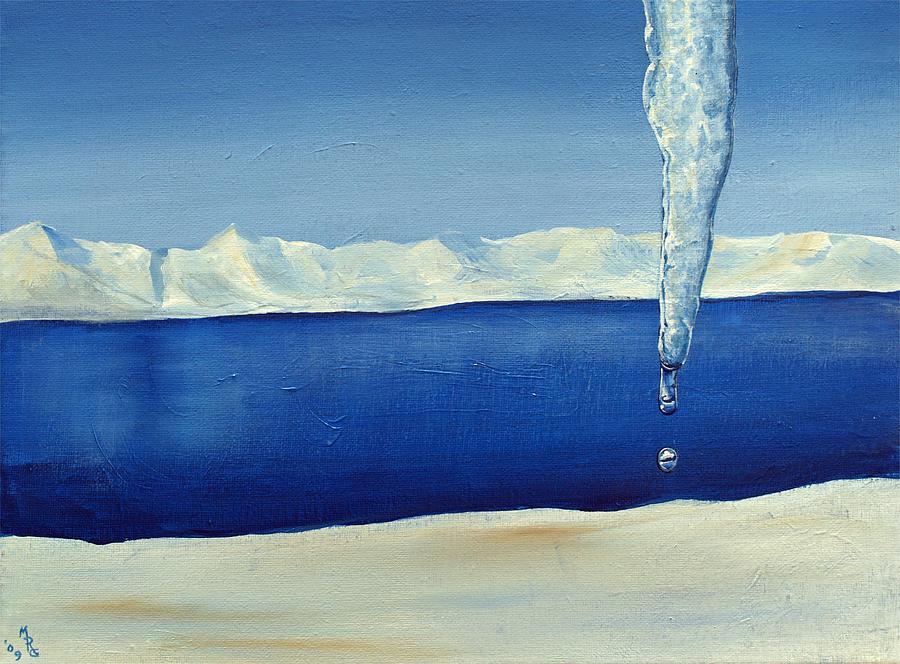The image is a modern art oil painting, signed by the artist with initials "MRC '09" in the bottom left corner, indicating it was created in 2009. The scene vividly depicts a glacial landscape, possibly inspired by regions like Antarctica or Alaska. The composition features a striking contrast of colors, dominated by shades of blue and white. The sky transitions from light blue at the horizon to a deeper blue towards the top, reflecting the cold atmosphere.

Central to the image is a deep blue lake with lighter blue ripples caused by a water spout rising from the right side of the lake. The lake's surface is further detailed with scattered water droplets, particularly noticeable in the lower-left corner. Surrounding the lake are snow-covered peaks and ice formations, adding to the frigid ambiance.

Notably, in the top right corner of the painting, a large icicle hangs down, appearing to drip as if it were melting, with visible water droplets adding to the realism. Along the upper edge of the painting, white and light blue glaciers stretch across the landscape, enhancing the feeling of a cold and desolate yet beautifully serene environment. The blend of sand-like textures and icy elements along the shoreline highlights the artist's intricate depiction of a glacial terrain amidst an expansive blue sky.